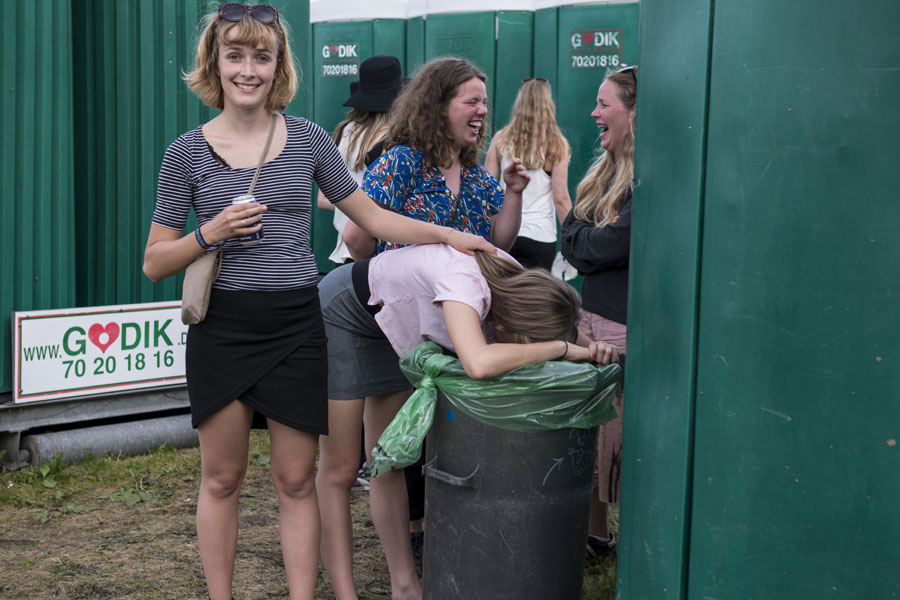This photograph, capturing a moment at an outdoor festival, features a young girl bent over a black rubber garbage can with a green bag, likely throwing up. She has light brown hair and is dressed in a short-sleeved pink shirt paired with a gray skirt. Her blonde-haired friend, about 16 or 17 years old, stands beside her, kindly holding her hair out of her face while smiling at the camera. The friend is adorned in a short-sleeved black-and-white striped shirt, black skirt, and has sunglasses perched on her forehead. Surrounding them are several green port-a-potties and festival attendees, including two women in the background who appear to be laughing heartily, showcasing their amusement. A white rectangular sign with green print reading "WWW.GODIK.D70-2018-16" is visible on the far left. The scene is vivid with elements such as the green port-a-potties and the contrasting outfits of the central figures, encapsulating a candid, yet somewhat unusual moment at the event.